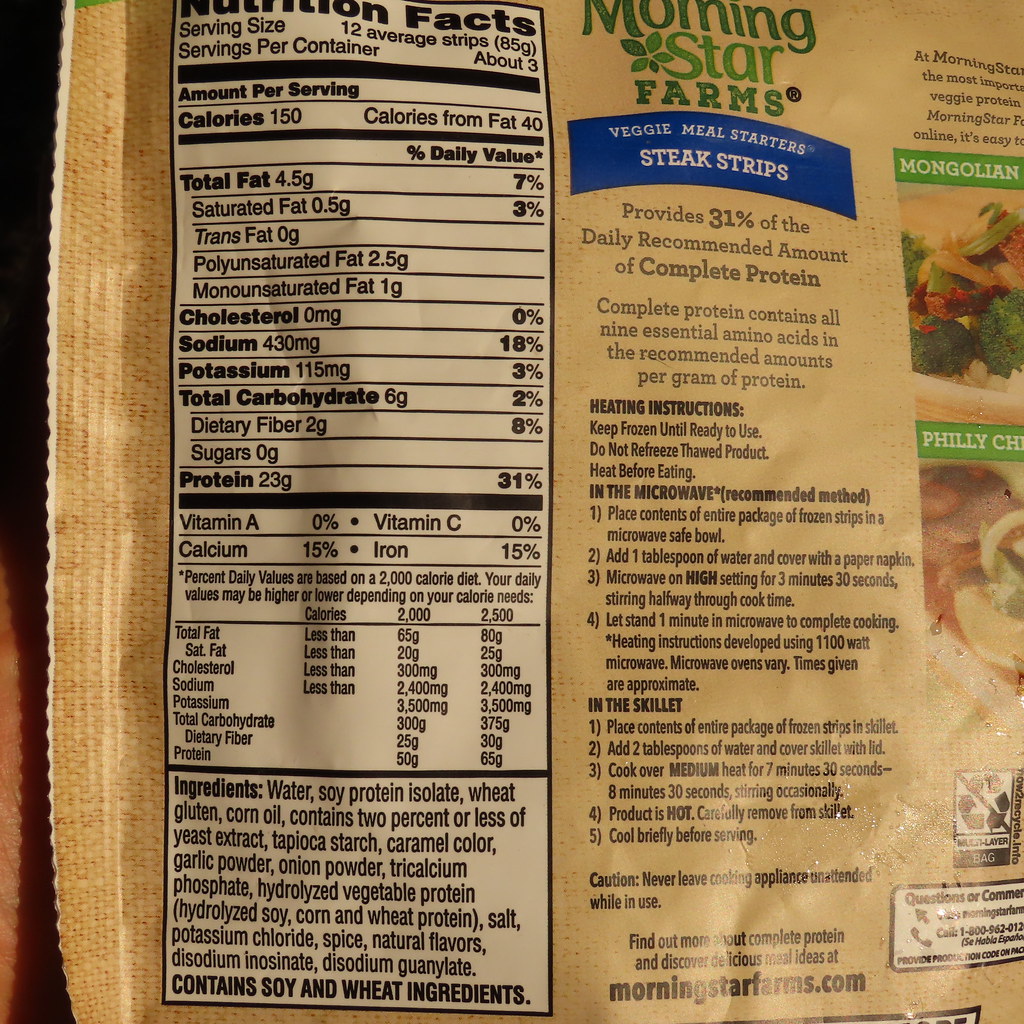This image showcases the back of a MorningStar Farms Veggie Meal Starter Steak Strips Frozen Meal Package, designed with a tan color scheme. Taking up the left side, prominently displayed, are the nutrition facts: serving size (12 average strips), servings per container (about 3), and the amount per serving with details such as calories, total fat, saturated fat, cholesterol, sodium, potassium, protein, sugars, and vitamins. Below these facts is an ingredient list including water, soy protein, wheat gluten, and corn oil.

On the right side of the package, below the MorningStar Farms logo, there's a note indicating the product provides 31% of the daily recommended amount of complete protein. Heating instructions for both microwave and skillet methods are detailed beneath, accompanied by a caution. There’s also a website link, MorningStarFarms.com, for further information.

Adjacent to this section, a partially visible image of mixed vegetables can be seen, with the words "Mongolian" at the top of this picture, followed by an image of onions captioned "Philly." There is also a box for questions or comments, and the package is marked as non-recyclable.